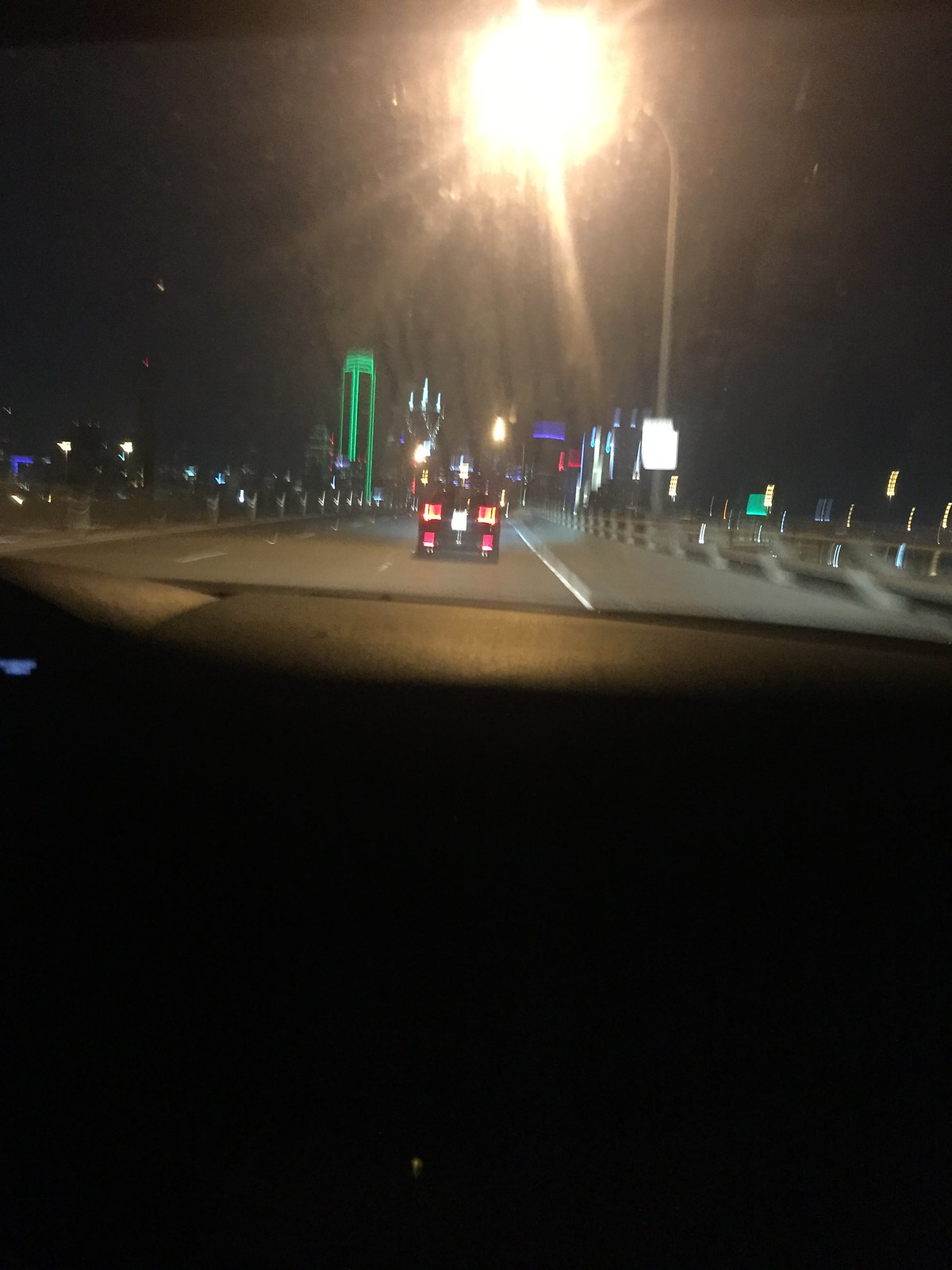The photograph captures a nighttime scene from the point of view of a driver inside a car. The image focuses on the road ahead, where a black vehicle's taillights are visible, driving along an illuminated street. The car appears to be on a bridge, as suggested by the visible railings on either side of the highway. At the bottom left of the image, part of the dashboard is visible, with bluish-purple lettering that is slightly out of focus. 

Above, a brightly lit street lamp casts a glow across the scene, further emphasizing the nighttime setting. The distant cityscape is dominated by buildings adorned with neon lights: one building is outlined in green, another features neon violet and neon red lights, and a third building showcases bluish lights forming a circle, with three poles of light at its top. Street signs and additional lamps add to the urban atmosphere, while the black sky forms a stark backdrop to the vivid, colorful lighting.